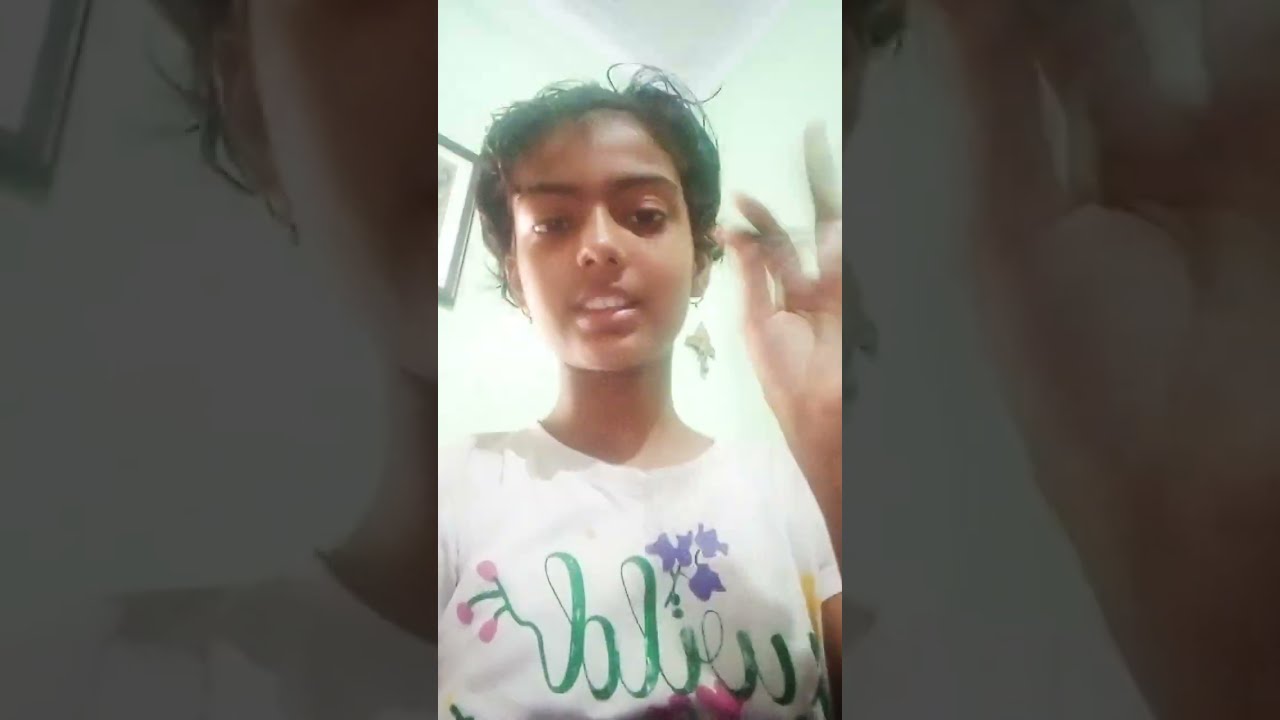The image features a young girl, likely around 15 or 16 years old, who appears to be of South Asian or Mediterranean descent with medium-toned skin, dark eyes, and dark, possibly short, hair that is either cut short or pulled back from her face. She appears to be smiling or talking, her mouth slightly open, revealing her top row of teeth. She is wearing a white shirt that has green cursive text integrated with pink and purple floral designs. The text on her shirt is somewhat fuzzy but suggests a word like "Valio." 

She is holding her left hand up, her thumb and pointer finger pinched together as if snapping or gesturing, and she is adorned with large earrings. The background reveals a white wall with a black-framed photograph and another decorative item, while a light mint green hue seems to accentuate the surroundings. 

Additionally, the photo has a unique aesthetic with grayed-out, enlarged border elements on either side, showcasing closer sections of her hand and face, creating a shadow-like effect that frames the main image.